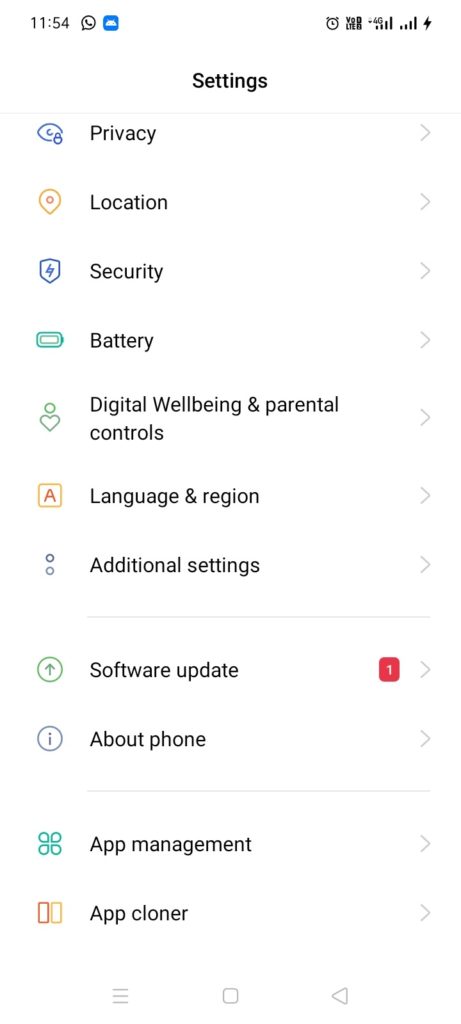In this image, we observe a smartphone interface displaying a variety of settings, applications, and informational icons. The time is prominently positioned at the top of the screen, accompanied by notifications, signal strength indicators, and a battery icon that shows the remaining charge. Each app and setting is marked with a recognizable icon on the left side, hinting at their functions. Toward the bottom of the screen, there are buttons for additional actions such as opening more options or returning to a previous page. This detailed layout provides quick access to multiple functionalities, allowing the user to navigate the device with ease.